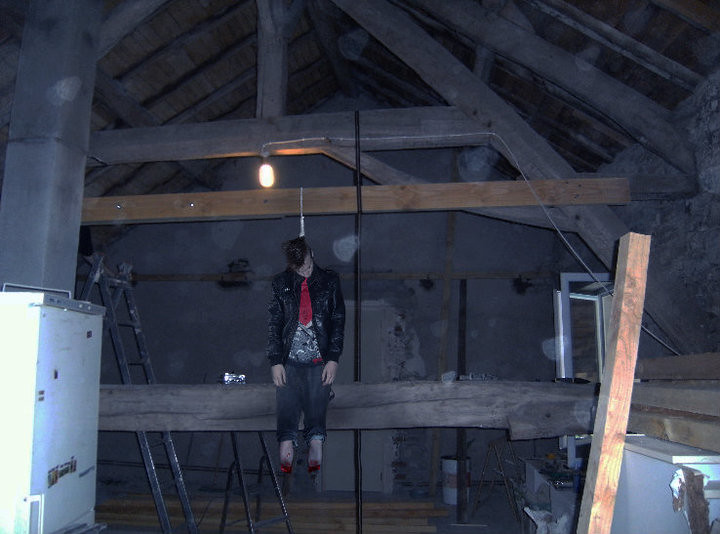The image depicts a grim scene in a cavernous, attic-like room with aged, stone walls and a wooden A-frame roof. Thick, dark wooden beams run horizontally across the room, and a large central beam serves as the anchor point for a noose. From this noose, a figure is hanging, dressed in a black leather jacket, a red t-shirt, and dark pants. The figure, which could be either a mannequin or a human, has bloodied stumps where its lower legs and feet should be. The complexion appears pale, almost grayish-white, suggesting further that it might be a Halloween prop or something similar for a horror setup. Scattered around are some pieces of wood and a ladder leaning against the left wall. A white unit, perhaps an electrical or heating device, is also visible to the left, beside a vent. Several orbs are noticeable across the room, possibly from dust or light reflections. On the right side, through the clear, white-framed window, natural light streams in, contrasting sharply with the dim, single bulb hanging directly above the suspended figure.